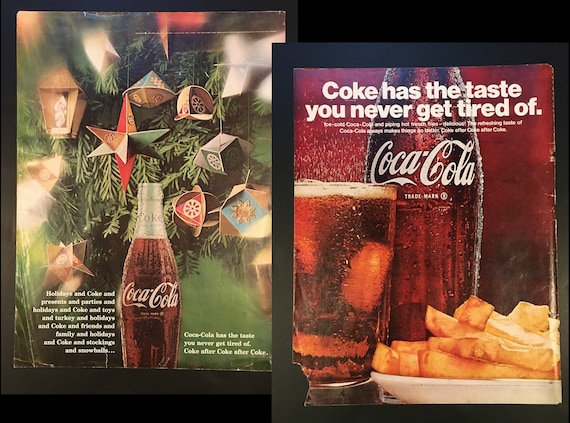This retro Coca-Cola advertisement features two vertical images side by side. The left image showcases a glass bottle of Coca-Cola in front of a decorated Christmas tree with various paper ornaments and boxed decorations. The label on the bottle has white writing, and the bottle appears wet, highlighting its refreshing quality. Accompanying the image is a festive slogan in a challenging-to-read white font: "Holidays and Coke, presents and parties and holidays and Coke, toys and turkey and holidays and Coke, friends and family and holidays and Coke, stockings and snowballs."

The right image, framed similarly to the left, depicts another glass bottle of Coke alongside a glass filled with ice and Coca-Cola, paired with a white dish of golden French fries. Above this image, bold white letters proclaim, "Coke has the taste you never get tired of." The overall design is completed with a nostalgic black frame surrounding each image, enhancing their vintage magazine ad appeal.